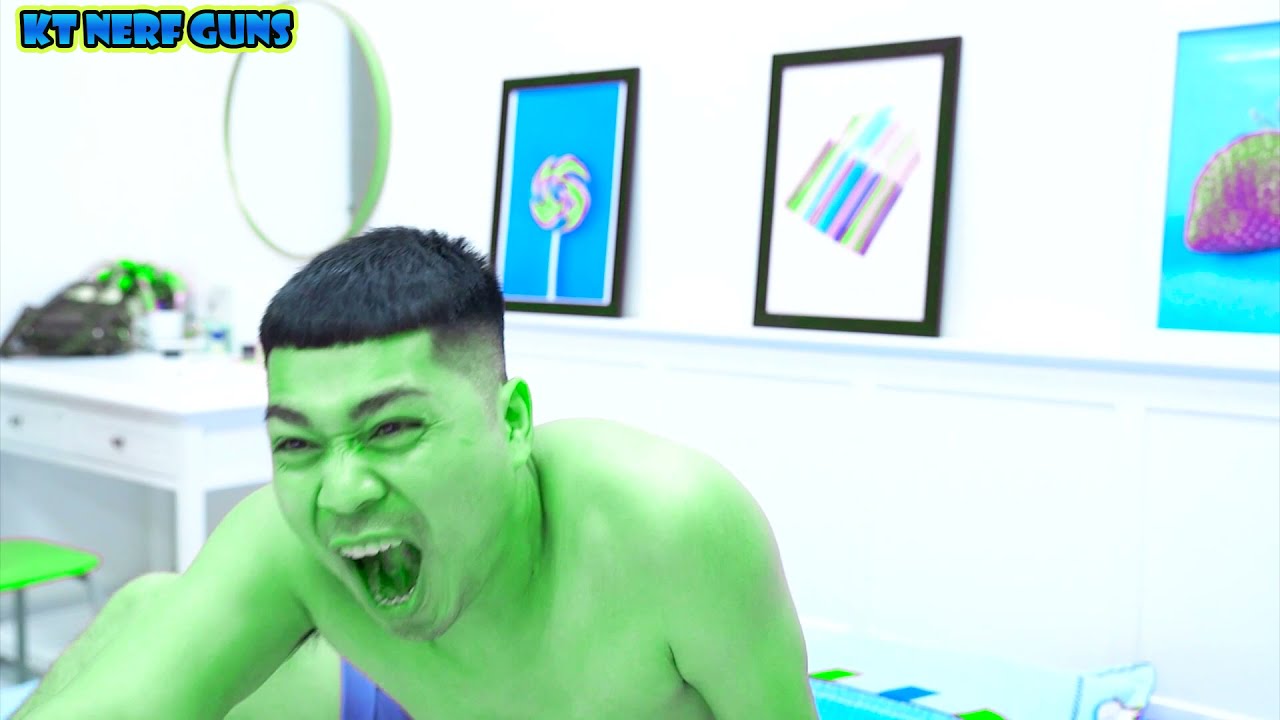The image depicts a young man with short black hair, painted completely in light green paint similar to the Incredible Hulk. He is shirtless and appears to be yelling, with his mouth wide open and intense wrinkles around his squinting eyes. He is facing downward towards the left, and one arm is extended in the same direction while the other hangs straight down by his side. His ear is painted the brightest green color, standing out against the rest of his green skin. 

In the background is a bedroom setting. Above him to the left, there is blue text outlined in black and yellow that reads "KT Nerf Guns." On the wall behind him, there are three framed pictures. One picture features a large candy cane, the second appears to depict markers, and the third one, which is farthest to the right, contains indistinct shapes in black, light teal, purple, and yellow. Additionally, there is a vanity with a mirror and a white desk visible on the left side of the image, with a green chair partially obscured in front of it. The photo captures the man's intense and animated expression, perhaps imitating the Hulk's anger.